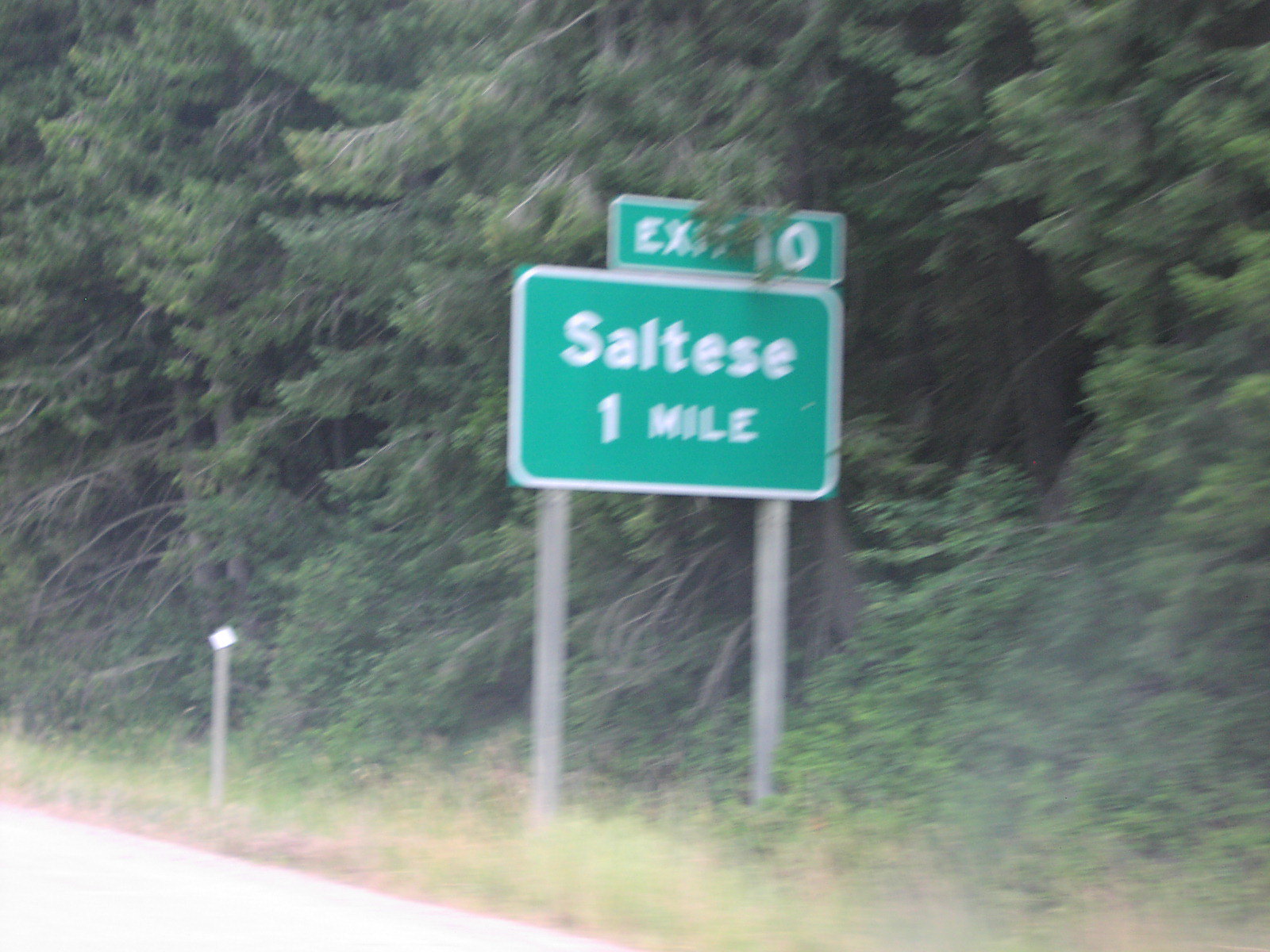This color photo, likely taken from a moving car due to the motion blur, captures a roadside scene featuring a standard green U.S. highway sign. The sign, mounted on two grayish posts, reads "Exit 10" on a slightly leaning rectangular plaque partially obscured by lush tree cover, and below it, "Saltice, 1 mile" in crisp white letters. Surrounding the road is a densely wooded area dominated by coniferous trees, primarily pines, with some openings where dead trees are visible. The foreground shows a strip of dirt right up against the roadway, which appears wind-swept with scattered dirt particles. A reflective roadside marker can be seen further beyond the main sign. The overall image has a slightly blurred quality, giving it a soft, less defined look.